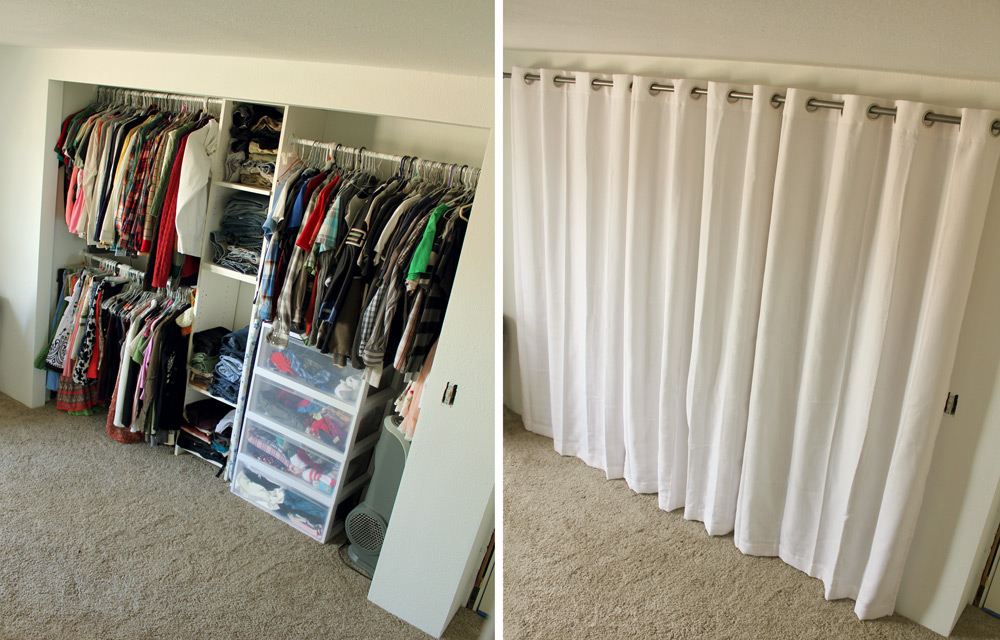The image is divided into two parts, presenting a before-and-after transformation of a closet space. On the left, the image depicts an open and cluttered closet with beige-tan carpet and off-white or cream-colored walls. The closet is tightly packed with various clothing items—likely indicating both male and female garments—hanging on three rods, two on the left side and one on the right. Accompanying the clothes are a clear plastic shelving unit or drawer unit, shelves holding sweaters or other articles of clothing, and possibly even a heater stored within. The door of the closet is either missing or folded back.

On the right, the same closet is now concealed by a large, white fabric curtain with pleats, drawn across a silver rod with large ringlets. This curtain completely covers the messy interior, giving the room a much neater appearance. A small, gold (or black) handle or connector might be present to aid in opening or closing the curtain. This transformation emphasizes the practical use of a curtain to hide clutter and create an organized look.